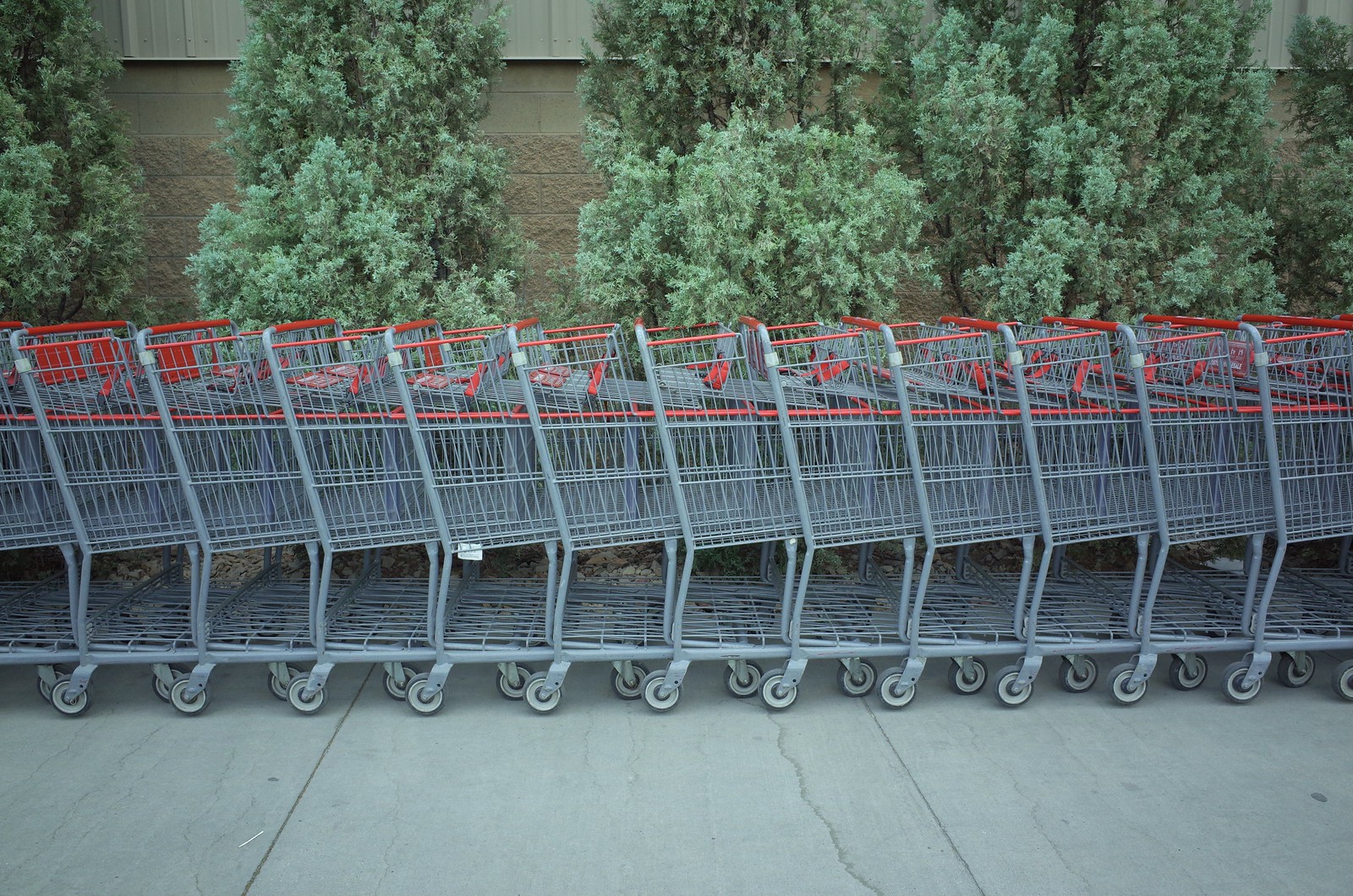This image captures a neatly arranged row of approximately 12 silver shopping carts with red handles and red child seats, standing on a cracked sidewalk. The carts, with their black wheels and white tags on the handles, appear new and clean. Behind them, a series of small, green trees, standing two to three times the height of the carts, partially obscure a brick building in the background. The carts are viewed from the side, lined up closely together as if recently gathered by a cart collector, and extend towards the right of the frame.